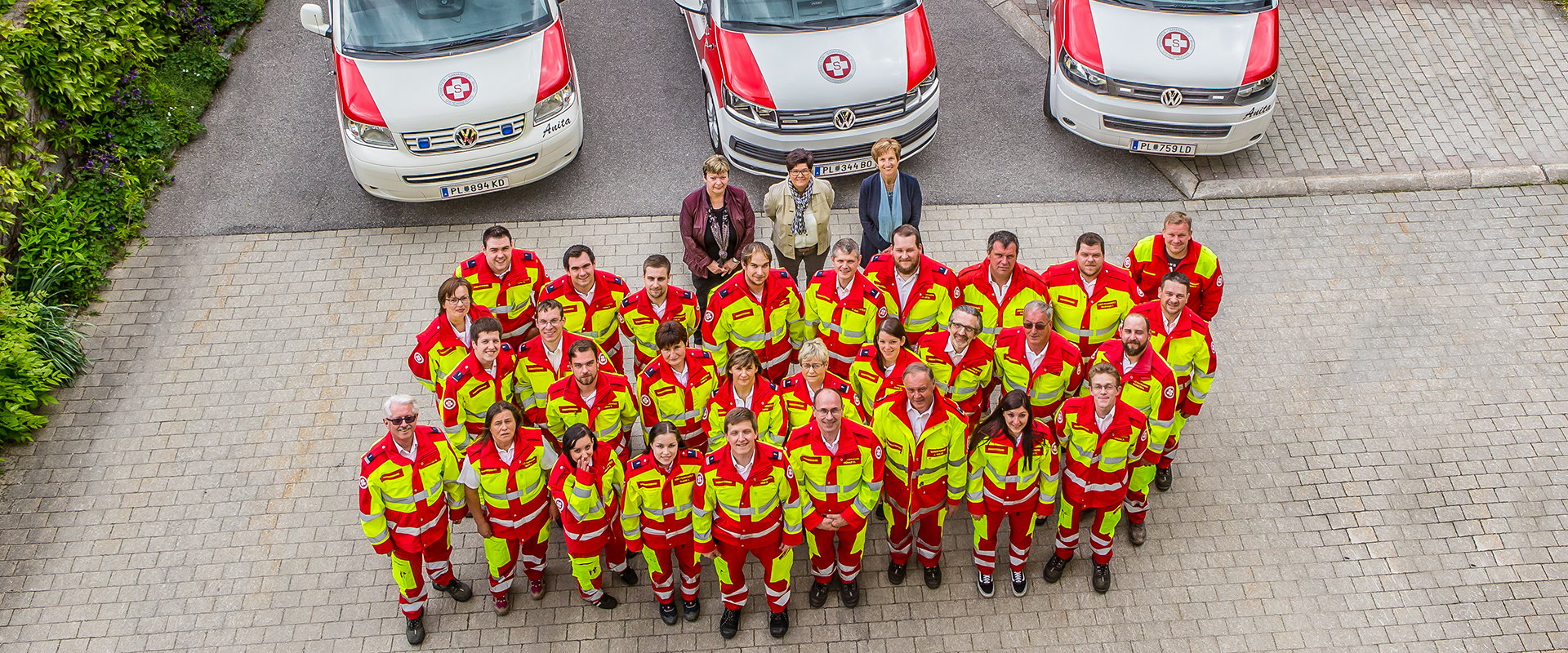This image is taken from an aerial perspective, showing a bustling scene centered around three ambulances, which appear to be VW vans, distinguishable by their European license plates and red fenders. The ambulances are parked on a mix of a gray cobblestone sidewalk and regular gray pavement. In front of the ambulances stand a large group of 30 to 40 people wearing matching yellow and red uniforms, likely indicating they are paramedics or firefighters. They are arranged in three or four rows and seem to be in high spirits, many of them looking up and smiling. Their footwear is predominantly dark-colored. Behind this group are three women dressed in business attire, potentially administrative staff, providing a contrast to the uniformed personnel. To the left, a cluster of bright green bushes adds a touch of greenery to the otherwise gray-toned setting. The scene captures a harmonious blend of emergency services personnel, administrative support, and their vehicles against an urban streetscape.